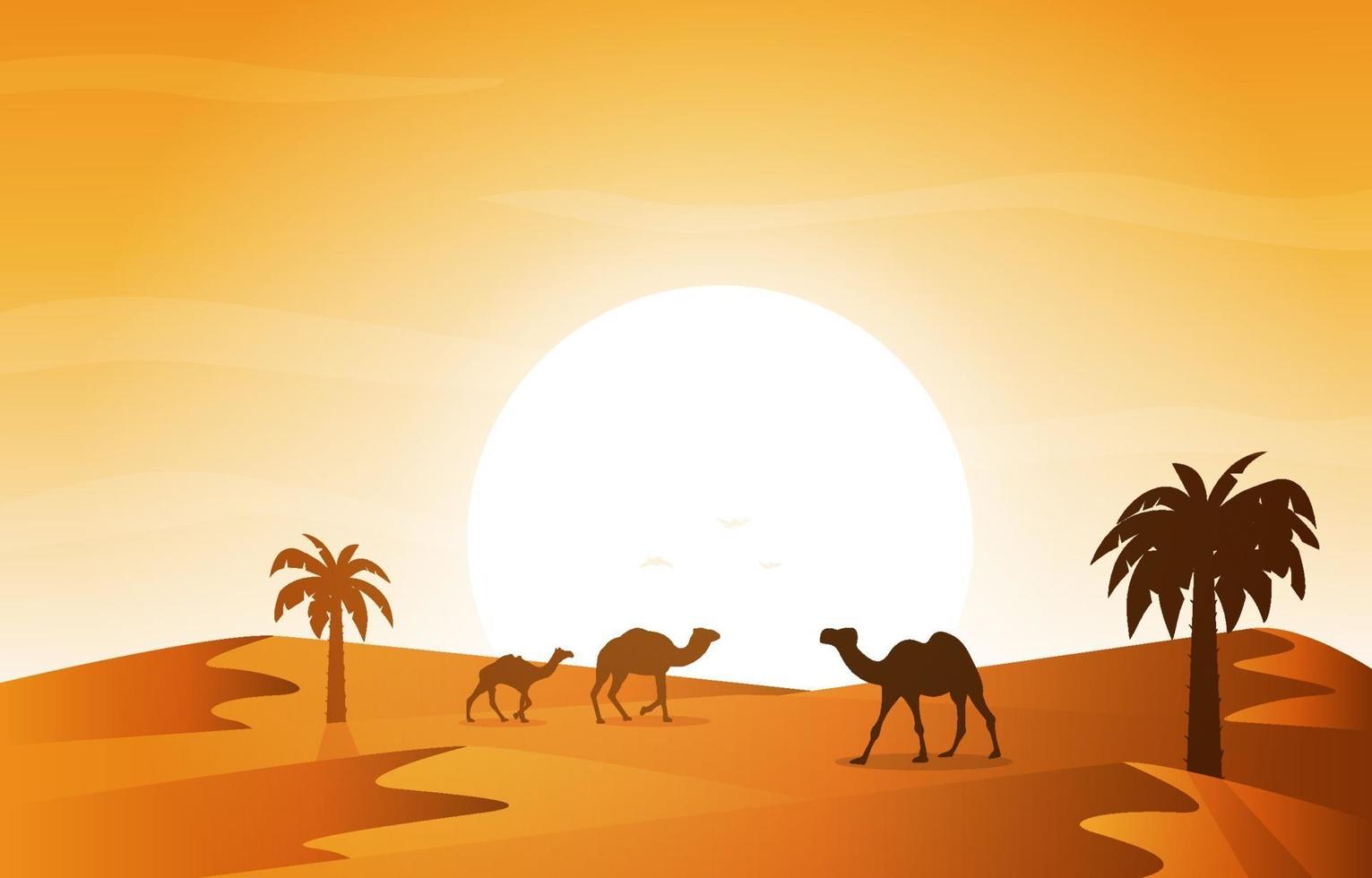This illustration depicts a desert landscape at either sunrise or sunset, characterized by its rich array of browns, golds, and light oranges. Dominating the scene is a large sun positioned just above the horizon, casting a radiant gradient of yellow and gold across the sky and sand. Below the sun, the foreground comprises rolling sand dunes, with their peaks forming a wavy, zigzag pattern, highlighted by dark brown and gold tones.

On either side of the composition, two palm trees stand tall, their silhouettes varying in size and color from brown to gold, contributing to the depth of the scene. Between these trees are three camels, positioned in such a way that their heads are silhouetted against the luminous sun. The camels differ in sizes, suggesting varying distances, with the smallest camel situated further away. Additionally, subtle details such as three small bird silhouettes can be discerned within the sun itself, enhancing the serene and slightly animated feel of the artwork. The sky above the horizon is interspersed with wavy white lines, likely representing clouds, adding texture and dimension to this enchanting desert vista.